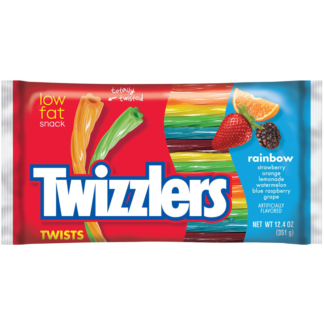This image displays a detailed package of Twizzlers licorice candy. The upper left-hand corner of the primarily red package reads "Low-Fat Snack" in yellow and white text. The central section is dominated by a large Twizzlers logo in white, outlined with a blue border for clarity. Below the logo, the word "Twists" is inscribed in smaller yellow letters. A clear wavy cutout in the middle of the package reveals multicolored Twizzlers inside—orange, yellow, green, blue, and purple. Adjacent to this window, the package features two Twizzlers, one orange and one green, with an arrow pointing to the orange one labeled "Totally Twisted." On the right side, within a solid blue column, images of an orange, a strawberry, and a blackberry emphasize the fruity flavors, all under text that reads "Rainbow." The intricate design and vibrant colors of the packaging emphasize the playful and varied nature of the product.